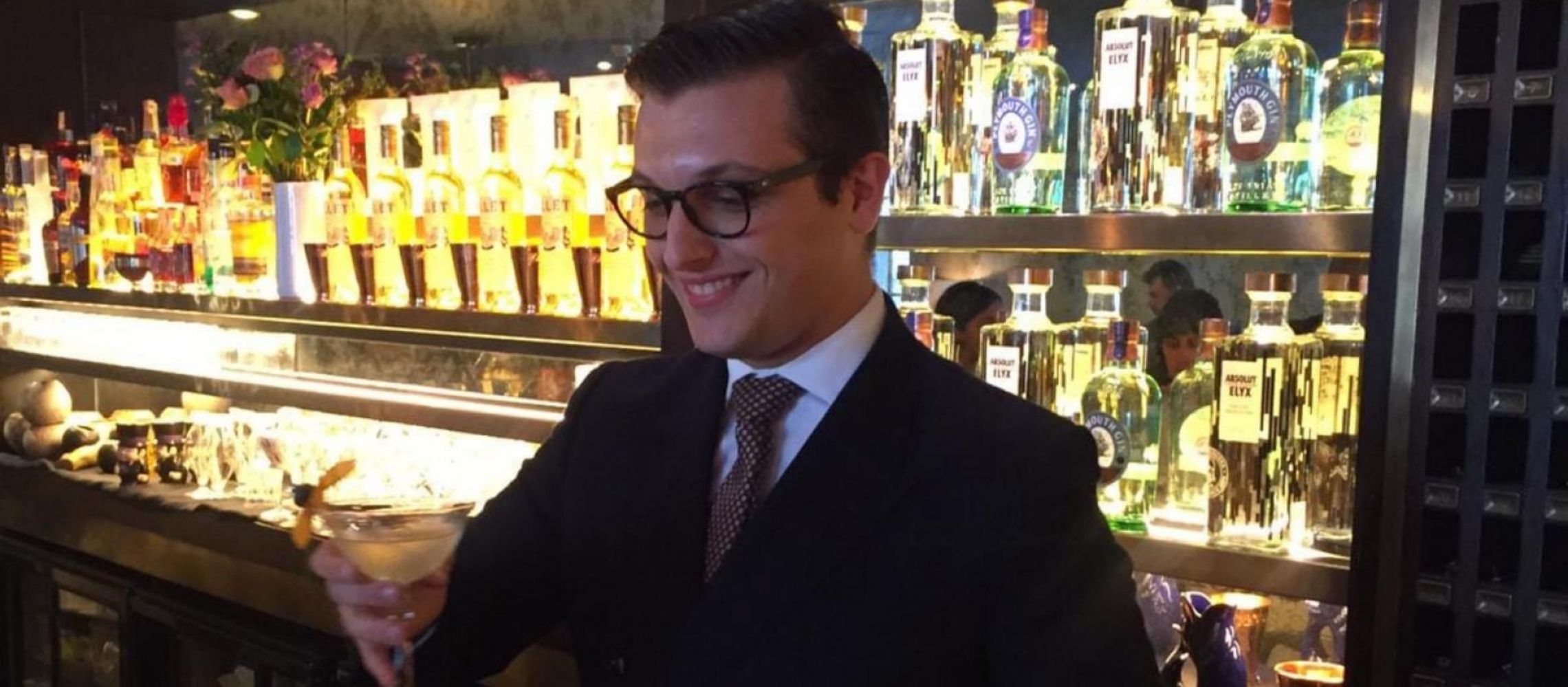The image depicts a young man in his late 20s to early 30s, who is smiling and wearing thick black-rimmed glasses and a neatly styled suit and tie with a white collar shirt underneath. Captured from the chest up, he is slightly turned to the left and looking down at a fancy cocktail in his hand. The cocktail glass is transparent with a flower garnish sticking out of it. Behind him, the bar displays an assortment of elegant liquor bottles, illuminated by a soft, golden light, creating a sophisticated ambiance. There are also some mixing glasses and possibly a register display nearby. Additionally, there are three faintly visible figures in the background, either as reflections or standing behind the shelves. To the upper left of the man, there's a basket of flowers, adding to the bar's refined decor.